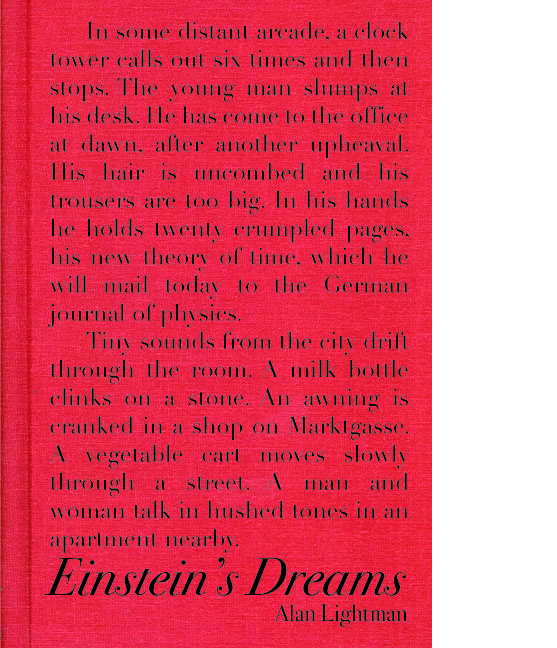The image is a portrait-oriented, rectangular book cover dominated by red and black colors. The red background is textured with weave lines, resembling an old hardback. At the top, black text in two paragraphs describes a scene: "In some distant arcade, a clock tower calls out six times and then stops. The young man slumps at his desk. He has come to the office at dawn after another upheaval. His hair is uncombed and his trousers are too big. In his hands, he holds 20 crumpled pages—his new theory of time, which he will mail today to the German Journal of Physics." The second paragraph reads, "Tiny sounds from the city drift through the room. A milk bottle clinks on a stone. An awning is cranked in a shop on Market Street. A vegetable cart moves slowly through the street. A man and woman talk in hushed tones in an apartment nearby."

At the bottom of the cover, in bold black print, the title "Einstein's Dreams" is prominently displayed, with the author's name, "Alan Lightman," in smaller print in the lower right-hand corner. The vintage print style contributes to a timeless, contemplative ambiance that captures the essence of the book.